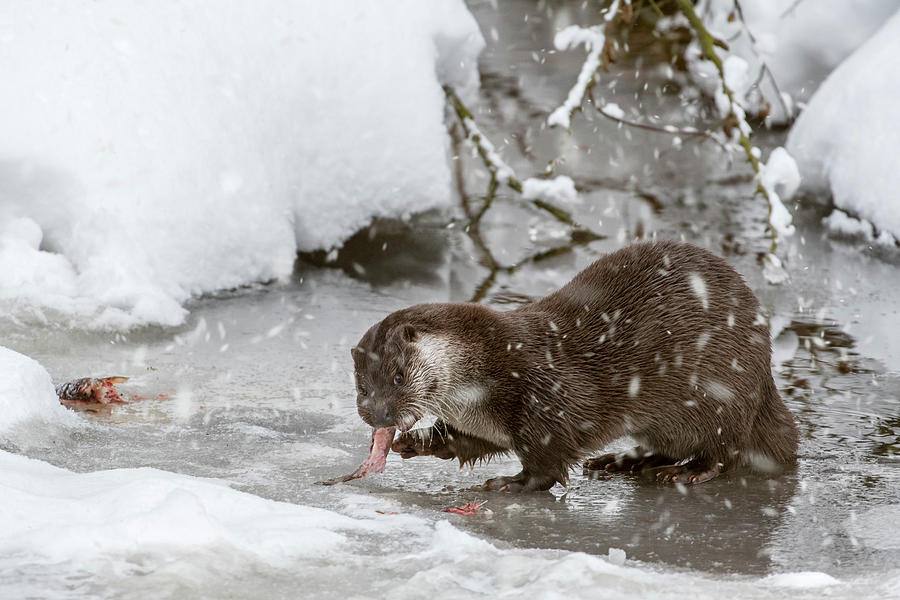This captivating winter photograph captures a lively brown otter with white markings on its chest, jaw, and cheeks, standing in a shallow, partially frozen stream. Amidst a gentle snowfall, the otter appears damp as it savors a pinkish fish, with a torn fish head lying on the ice to the left. The surrounding scene features snowy banks in the upper corners and snow-dusted tree branches arching above. The icy conditions extend throughout the stream, accentuating the cold, serene atmosphere of this wintry outdoors.